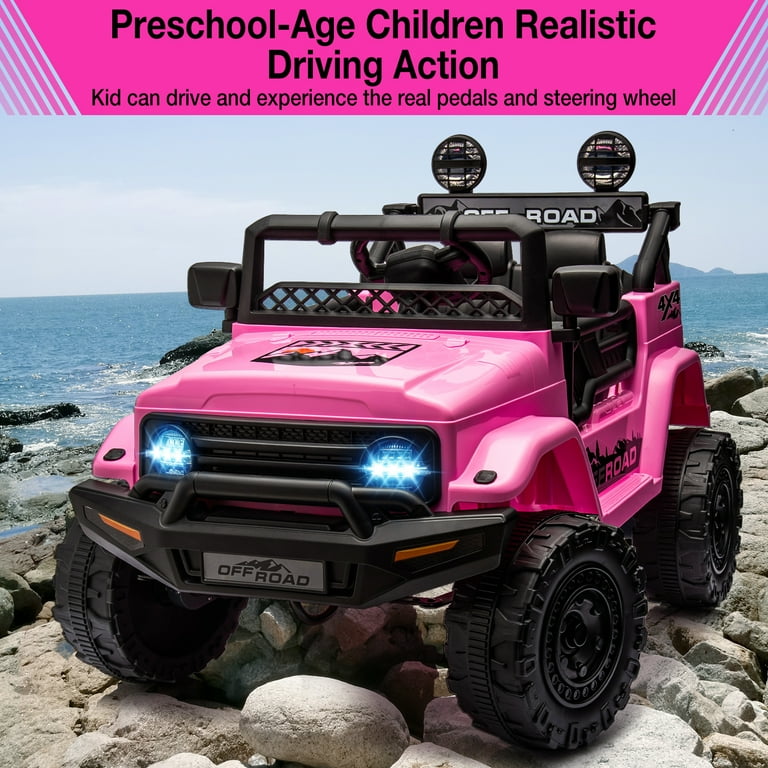This detailed photo captures a children's motorized jeep, depicted in a vibrant hot pink color with contrasting black wheels, black seats, and black accents. The jeep, which is a convertible with rugged, all-terrain wheels, is parked on a rocky beach. Its bright blue headlights are directed towards the camera, illuminating its license plate that cheekily reads "Off-Road Aunt." Adding to its playful allure, there's a sign on top of the jeep that states, "Preschool age children realistic driving action. Kid can drive and experience the wheel pedals and steering wheel." Behind the jeep, the scene transitions into a picturesque view of the ocean or a large lake, with foamy white water near the shore and various shades of blue extending toward the horizon beneath a clear, light blue sky.